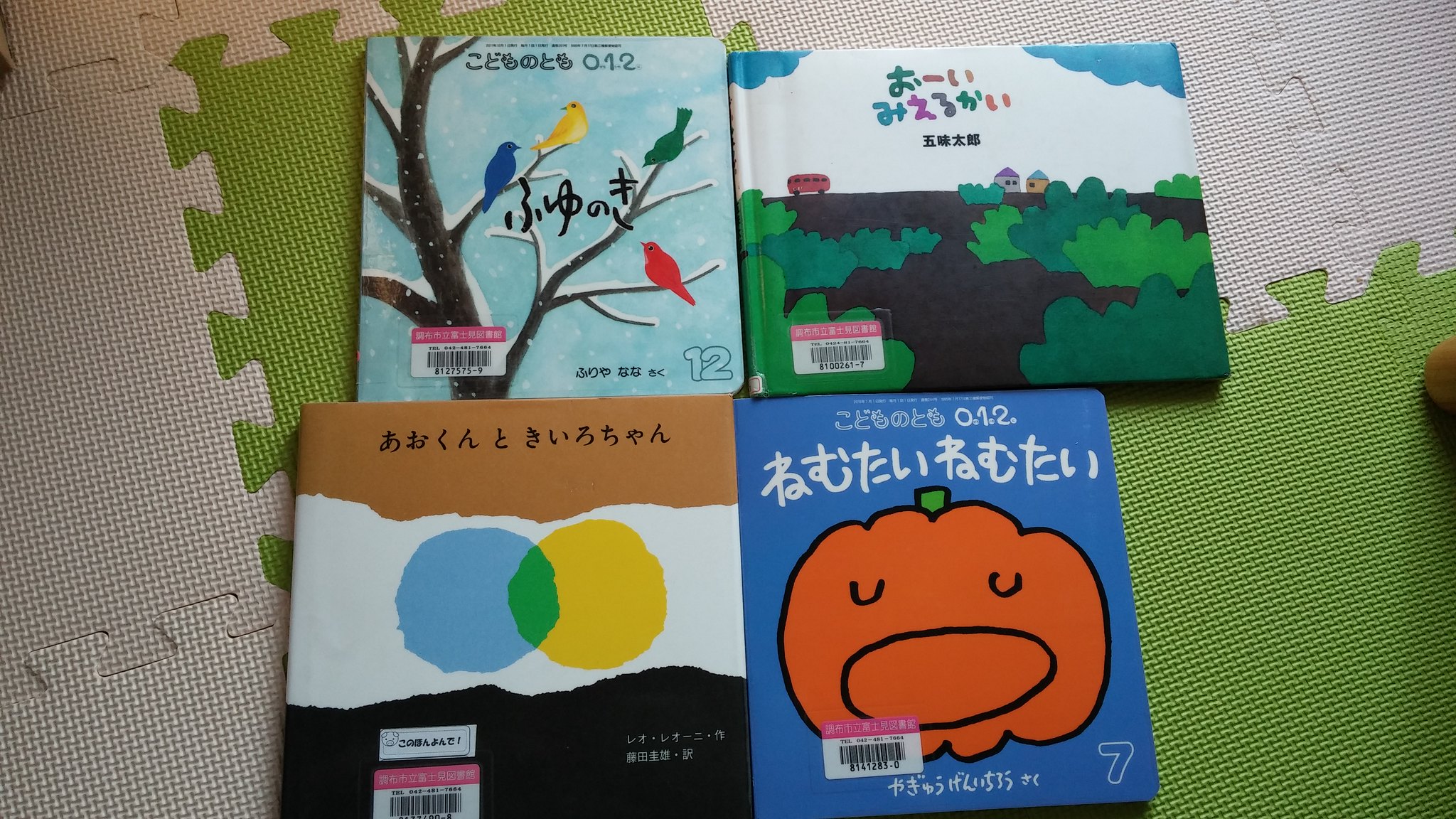This photograph showcases four children's books arranged in a square formation on a white and green, puzzle-shaped foam mat, reminiscent of a play mat typically found in a children's room. The books feature text in an Asian language, most likely Chinese or Japanese, and each cover depicts a different, vibrant design. The top left book displays a wintry tree devoid of leaves, with colorful birds perched on its branches against a light blue background. The top right book illustrates a whimsical landscape with a small bus and a couple of houses. The bottom left book features a bold pattern with three horizontal stripes—brown at the top, white in the center with overlapping blue and yellow circles forming a green ellipse, and black at the bottom. The bottom right book presents a large orange pumpkin with its mouth open on a blue background, resembling a sleepy visage. Each book bears a sticker tag with a UPC code or a red title, further emphasizing the organized yet playful aesthetic of the scene.